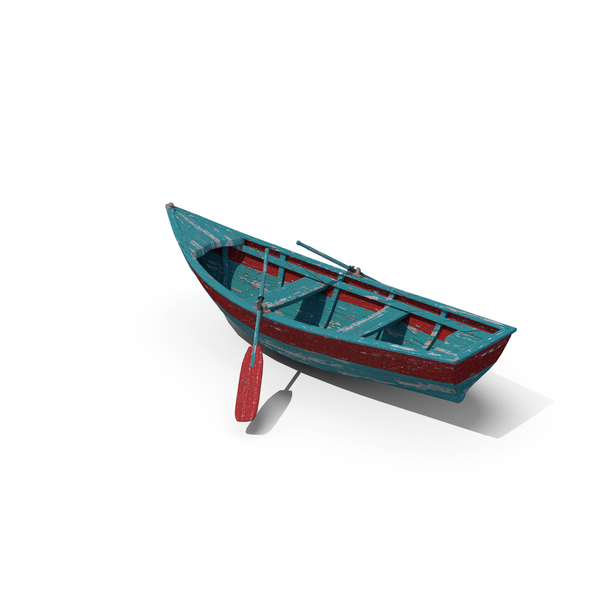Against a stark white background, the image features a weather-beaten, teal-colored wooden canoe. The exterior and interior of the canoe are adorned with a distinctive dark red stripe just beneath the gunwale. The paint on the boat is peeling, revealing gray patches of bare wood underneath, signifying age and extensive use. The canoe is equipped with two pairs of oars; one pair on each side. The oar on the bottom left distinctly shows a teal handle and an orange paddle, while the other oar's teal handle is visible sticking up on the opposite side. The boat has two wooden boards crossing the interior - one centered between the oars and another positioned slightly behind it. The canoe narrows to a point at the front and has a flat rear. Although it's suspended in mid-air, both the canoe and the oars cast subtle shadows beneath them, adding a touch of depth to the otherwise plain background.